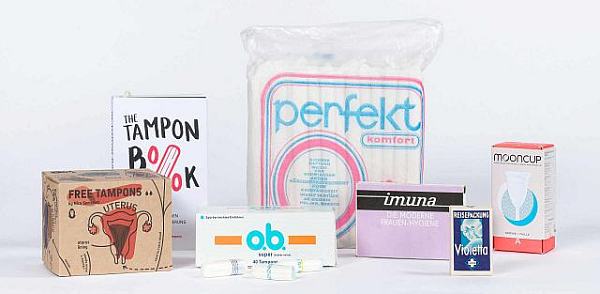The photograph showcases an array of seven different feminine hygiene products arranged on a flat white surface with a minimalist white background. Starting from the left, there is a brown square-shaped box labeled "Free Tampons" with an illustration of a uterus. Behind this box, there is a hardcover book titled "The Tampon Book" with a white cover and black text. To the right of the book, there is a white rectangular box labeled "OB," appearing to be another box of tampons. Behind the OB box, prominently placed in the center, is a large transparent plastic bag labeled "Perfect Komfort," filled with tampons. Directly in front of the OB box, there are some smaller tampons that have seemingly spilled out. Moving further to the right, there is a box labeled "Immuna," followed by a smaller box labeled "Violetta." At the very end, there is a box labeled "Moon Cup," featuring a drawing of a menstrual cup. The overall impression is that this image could be an advertisement or a display showcasing the variety of available feminine hygiene products. The photograph has an old, compressed quality, adding a vintage feel to the composition.